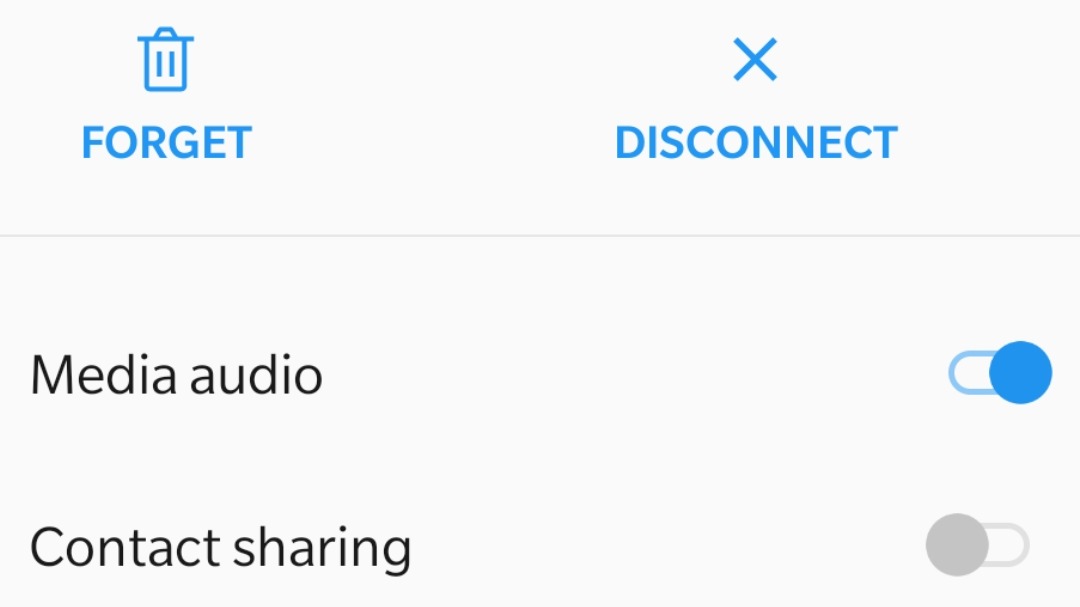The image features a white background with settings for a device displayed prominently at the center. At the top, "FORGET" is written in large, bold, blue capital letters, accompanied by an illustration of a garbage can. Below that, "DISCONNECT" is similarly displayed in blue and is marked with a large "X". Underneath these headings, the setting "MEDIA AUDIO" is written in bold black text and is highlighted in blue, indicating it is selectable. Below "MEDIA AUDIO", the setting "CONTEXT SHARING" is displayed, with a gray "OFF" button indicating it is currently disabled. The settings are encapsulated in a gray box, emphasizing the contrasting bold letters and buttons. The image is straightforward, focusing solely on these specific device settings, without any additional context or information.